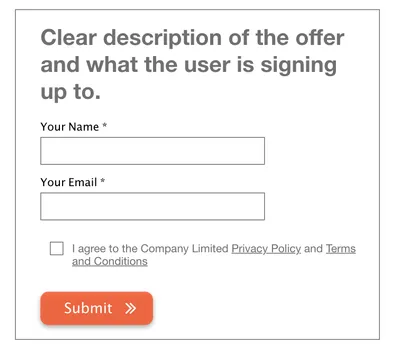The image is a screenshot from a website, depicting a sign-up form area encased by a light to medium gray square border. Within this square, there is a clear description of the offer in a prominent position, with the word "Clear" starting with a capital 'C'.

Below the description, two input fields are displayed sequentially. The first field is labeled "Your Name" (with 'Y' and 'N' capitalized), followed by an asterisk, indicating a required field. This is accompanied by a blank space provided for the user to input their name. The second field is labeled "Your Email" (with 'Y' and 'E' capitalized), also marked with an asterisk and a blank space for email input.

Further down, aligned slightly to the right, there is a checkbox followed by the sentence, "I Agree to the Company-Limited Privacy Policy and Terms and Conditions." In this sentence, 'Company' and 'Limited' are capitalized, and both "Privacy Policy" and "Terms and Conditions" are underlined, with each word starting with a capital letter, indicating clickable links to detailed documents.

Finally, at the bottom, there is a prominent orange submit button with the word "Submit" written in white text.